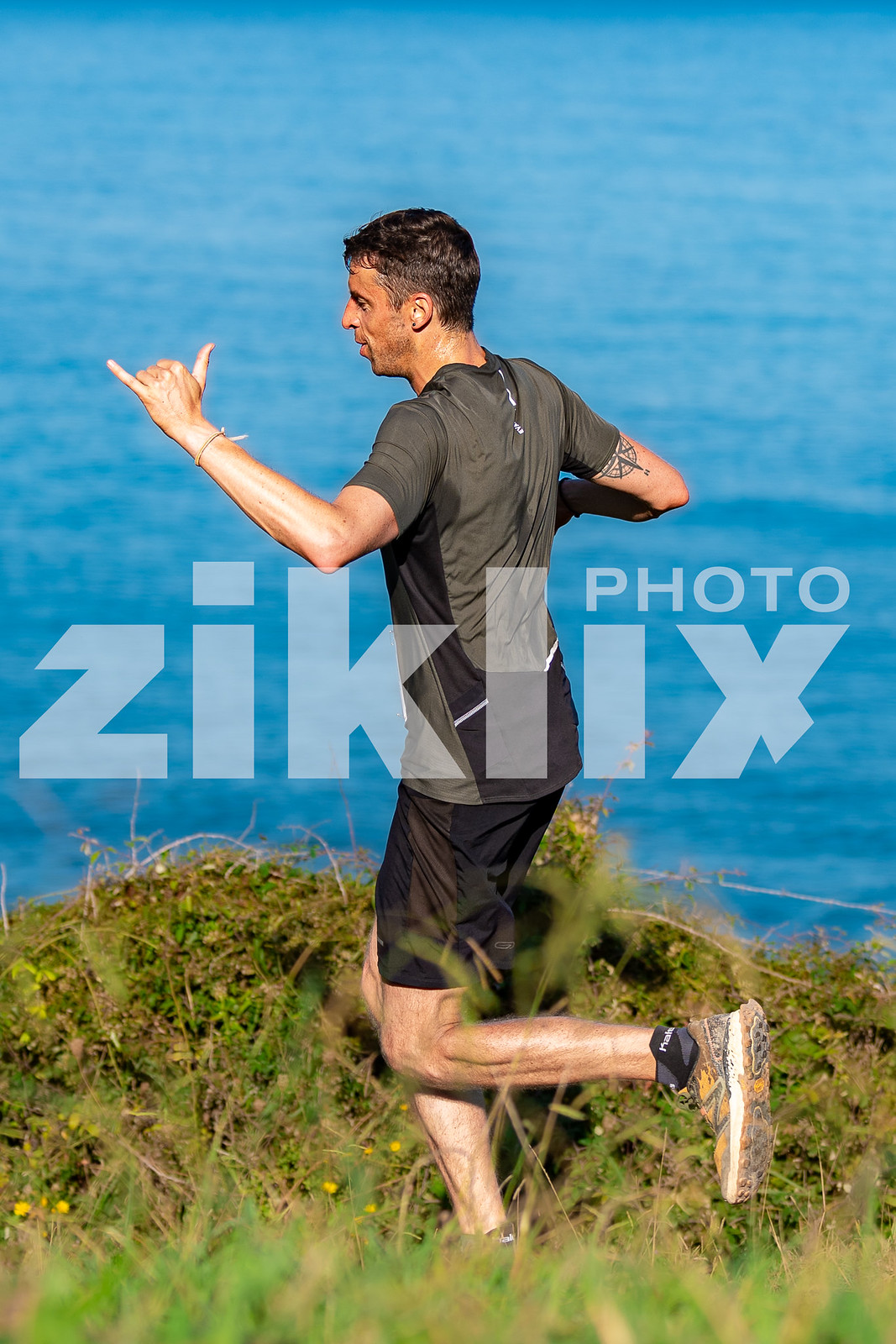The photograph features a muscular man running on a grassy hill with a blurred grassy foreground dotted with yellow dandelions. The man, with short black hair and a medium golden skin tone, is captured mid-stride, facing left with his left foot in the air and right on the ground. He is dressed in black shorts, a dark gray short-sleeve shirt, and yellow running shoes with black ankles and white outer soles. His left arm, bent at the elbow with the thumb and pinky extended upwards, shows a barely visible tattoo. In the distance, a blue body of water, likely part of the ocean, forms the backdrop, adding a serene quality to the dynamic scene. Over the center of the image, the semi-transparent text reads "photo Ziklix" in a grayish-white font.